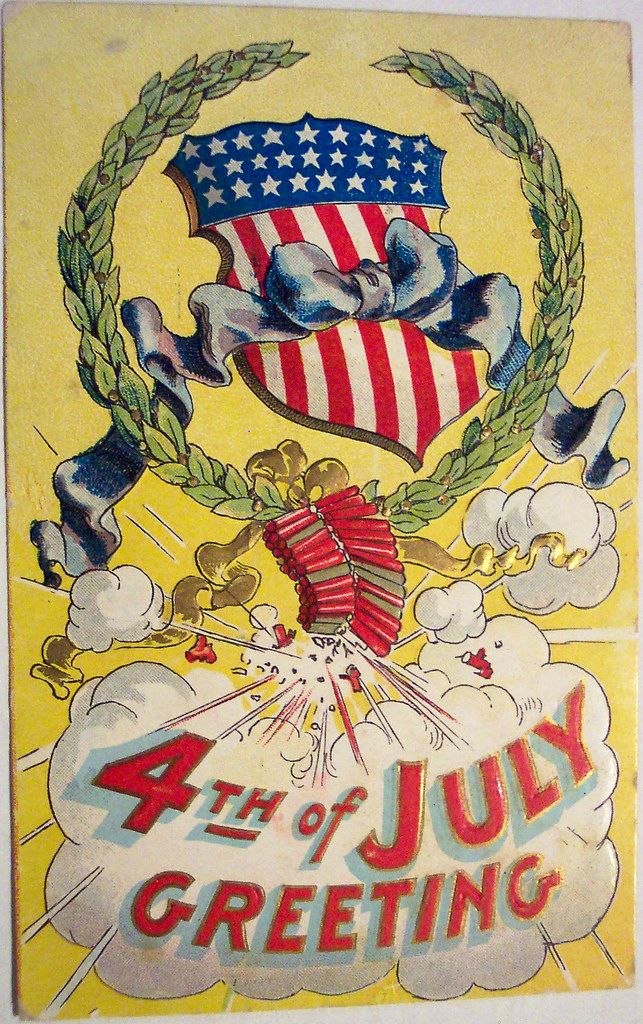This vintage-style poster, slightly faded and reminiscent of an old-fashioned postcard, celebrates the American Independence Day, the 4th of July. Dominating the top portion of the image is a crest in the shape of a shield patterned with the American flag. The flag design features blue and white stars at the top of the shield, while red and white stripes occupy the lower portion. A blue ribbon, tied in a knot, elegantly drapes across the shield. Surrounding the shield is a green laurel wreath, adding a touch of classic decorative flair. 

Below the wreath, a cluster of red and brown firecrackers dangles, their explosions forming clouds of smoke. One larger smoke cloud prominently displays the "4th of July greeting" in red font, capturing the festive spirit of the holiday. The background of the poster is a warm, vintage yellow, enhancing its nostalgic appeal. Overall, the image conveys a rich, celebratory ambiance with its blend of patriotic symbols and vintage aesthetics.